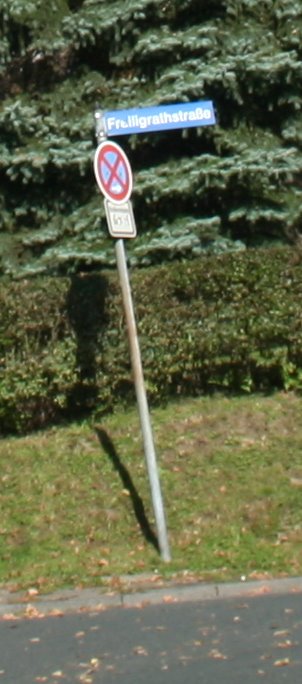This photograph captures a street sign situated in a foreign country, indicated by the unique name "Fralligatosstradle" jutting out prominently from the post. Below the street name, there is a double red "X" crossing out another sign, implying something is restricted or prohibited. Further down, additional information is displayed on the post, although it's not explicitly detailed in the description.

The street sign is mounted on a pole positioned adjacent to the street and curb. The landscape around the sign features a slight upward grade covered with grass, leading to a well-trimmed hedge. Beyond the hedge, the bases of tall fir trees are visible, suggesting an expansive wooded area in the background. The overall setting provides a blend of urban and natural elements.